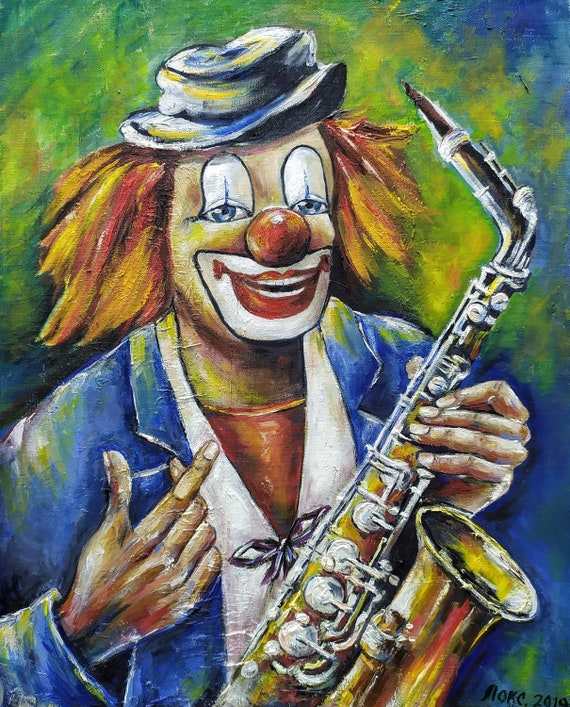This is an oil painting titled "Mocha 2018" that depicts a jazzy clown playing a saxophone. The clown is positioned in the center of the image, holding a gold saxophone with silver keys in his left hand. The clown appears joyful, with a smile on his face, his right hand extended with the index finger raised. He has bright red, frizzy hair topped with a hat, and is adorned in traditional clown makeup featuring a big red nose, exaggerated red lips surrounded by a white circular shape, and jester-like designs over his eyes. He is dressed in a blue jacket speckled with green patches, and a white shirt. The background is a vibrant patchwork of blue and green hues, adding to the whimsical atmosphere of the scene.